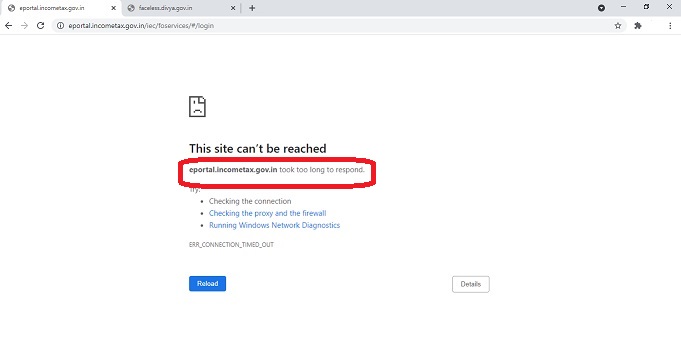The image depicts a Chrome browser window with two open tabs, both attempting to access the Indian government’s income tax e-portal. The user is currently on the first tab, where they have tried to navigate to "eportal.incometax.gov.in," but have encountered an error page stating, "This site can't be reached." The URL provided took too long to respond, suggesting issues such as connectivity problems, proxy and firewall settings, or the need for running Windows diagnostics. Below this error message, there are two buttons: "Reload" and "Details."

The other tab appears to show a similar issue while accessing a different page of the same site, indicated by the partial URL visible in the address bar which reads, "/services/login." This suggests the user was trying to log in or access specific services on the government site. The webpage has a white background and a minimalistic design, emphasizing functionality over aesthetics. This situation is portrayed to highlight possible challenges in determining whether the connectivity issue lies with the user’s network or the server.